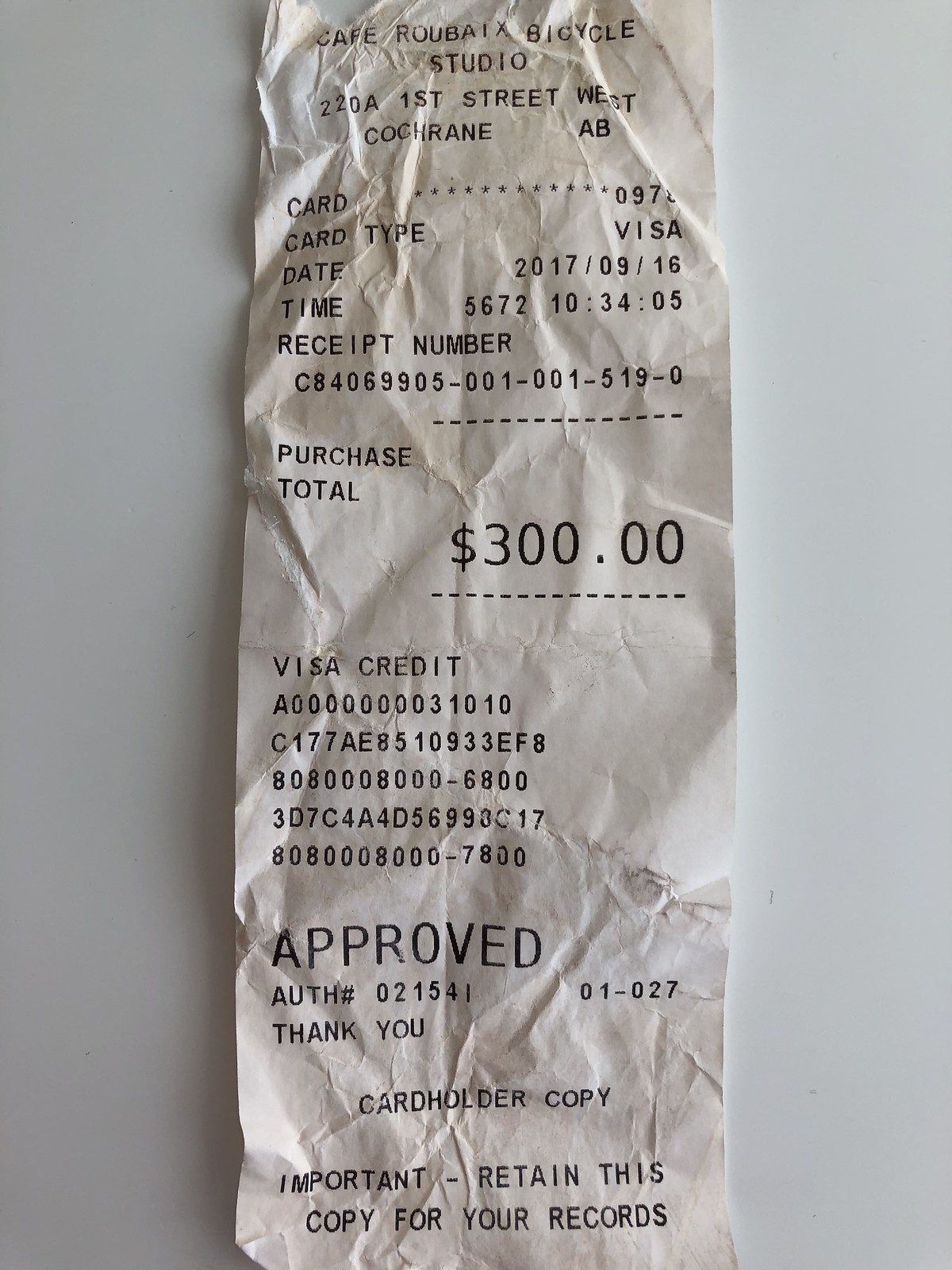This is a photograph of a crumpled receipt from Cafe Roubaix Bicycle Studio, located at 220A, 1st Street West, Cochrane, AB. The receipt is white with black writing, all in capital letters. The details on the receipt include: Card 097 (partially unreadable), Card Type: Visa, Date: 2017-09-16, and Time: 10:34:05 (format appears irregular as 05672-10-3405). The receipt number is C84069905-001-0015190, and the purchase total is $300. Payment was made via Visa Credit with a card identified by A0000000031010 with associated numbers C177AE8510933, EF880800080006800, 3D7C4A4D569936, and C1780800080007800. The transaction was approved with authorization number 08154107027. The receipt ends with a "Thank You" note, indicating it is a cardholder copy, with a reminder to retain the copy for records.